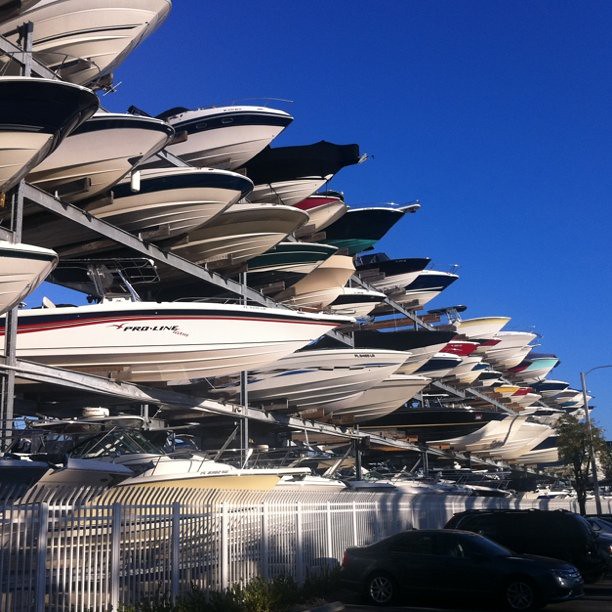The image depicts a marina boat storage area with multiple rows of boats stacked on four shelves, arranged from the largest on the bottom to smaller ones on top. The boats, varying in types and colors, including some with red and black stripes, predominantly appear white. One boat is identifiable with the name "ProLine" and an image of a bird on it. These boats, likely stored for the winter, suggest a secure facility rather than a store. A white fence with deterrent spikes surrounds the area, and to the right of the fence, there is a parking lot with three black cars, one small and the others larger, backed in near a light pole and a small tree. The sky above is a deep, rich blue with no clouds in sight.